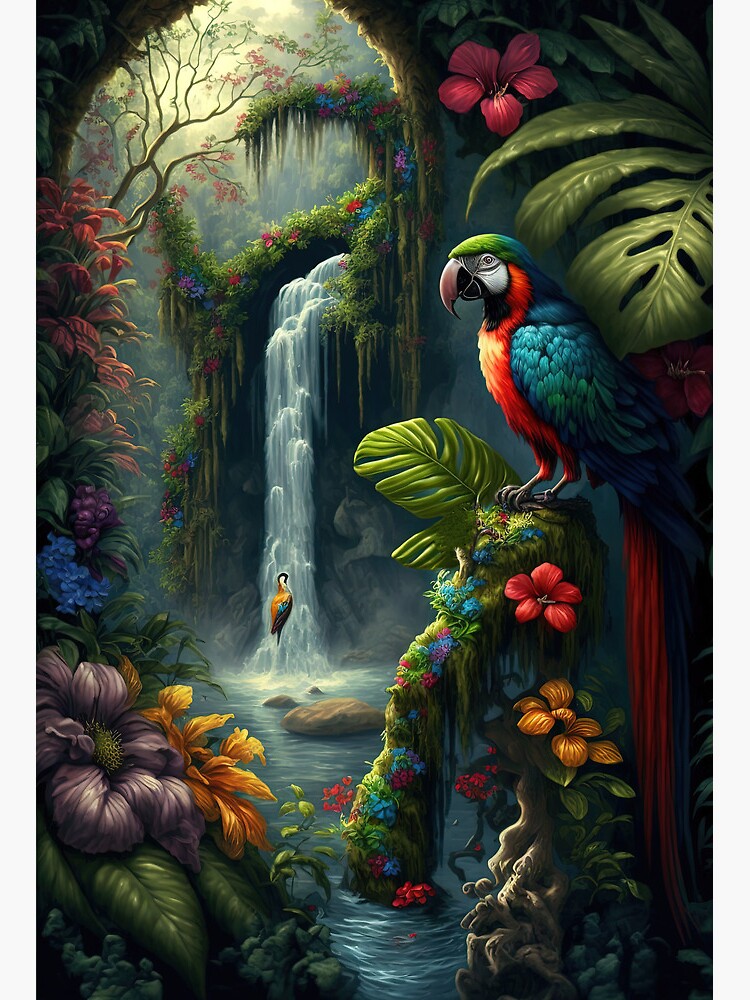This image is a vibrant and detailed scene that appears to be either a painting, drawing, or digital creation, showcasing an exotic paradise reminiscent of the Amazon rainforest. In the right-center of the image, a colorful parrot takes the spotlight. The parrot boasts a lime green head transitioning into deep ocean blue mixed with various shades of green and blue. Its curved beak is light pinkish, and it has a striking red neck and underbelly. The wings display a mix of blue and green feathers, while its tail features a combination of red and blue feathers. This parrot is perched amidst lush greenery and vibrant flowers, including purples, golds, reds, and blues.

Additionally, in the background, another bird, resembling a peacock with gold and pink feathers, can be seen standing underneath a cascading waterfall. The waterfall flows into a serene water body, surrounded by rocks and blooming flowers on the banks. The upper left-hand corner of the image depicts a sunlit area with yellow hues filtering through the dense foliage of the trees. The upper right-hand corner showcases more leaves adorned with a pink flower. Overall, the scene is filled with lush greenery, flowers, and an intricate canopy of trees, creating a vivid, almost Eden-like atmosphere.